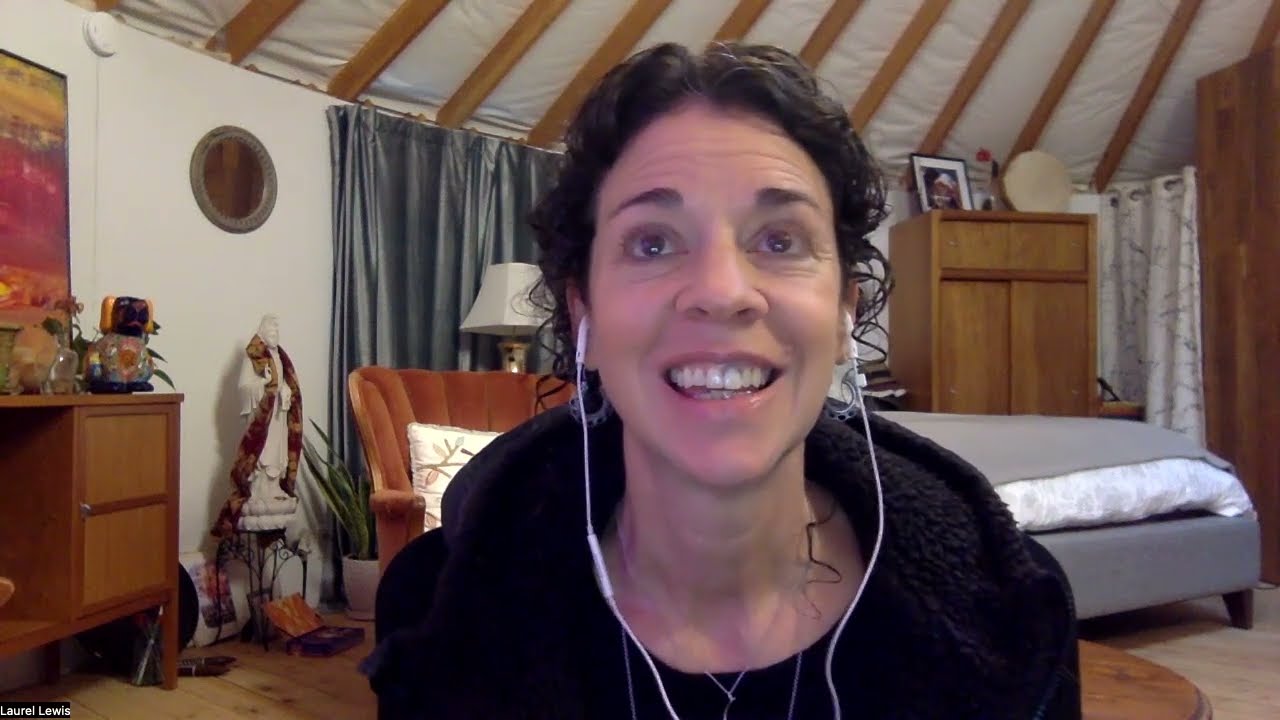In the center of this horizontal rectangular color photo is a smiling woman with a light complexion, wearing white wired earbuds. Her dark brown, curly hair cascades down to her neck, with long, thin spirally bangs framing her face. She’s dressed in a black, fluffy hooded jacket over a black top, adorned with delicate silver necklaces. She sits facing slightly upwards, appearing to be teleconferencing or streaming.

The background reveals a room with a distinct aesthetic. The ceiling features wooden rafters covered with white fabric. The walls are white, and a window is draped with gray curtains. To the left, there is a tidy desk cluttered with various objects and a colorful picture hanging above it. Behind the woman, positioned to the right, you can glimpse a round wooden table and a larger light-wood dresser or cabinet. Also visible is a bed with gray and white bedding, and a brown chair accentuated with a white throw pillow. The cohesive mix of these elements crafts a cozy and dynamic setting around her.